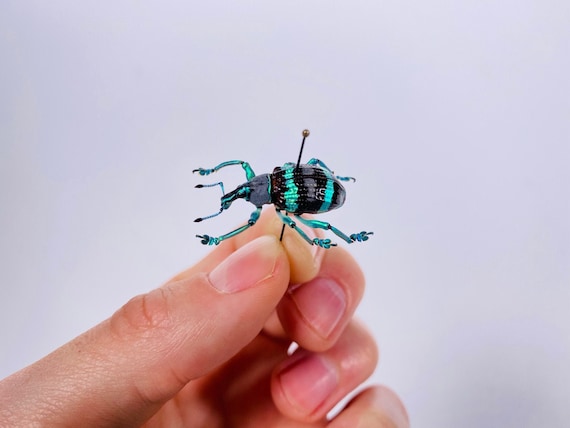The photograph depicts a hand with pale skin grasping a bobby pin between the thumb and index finger. The bobby pin impales a brightly colored beetle through its midsection. The beetle's body features a striking metallic blue-green iridescence intermixed with black stripes, and its L-shaped antennae emerge from its slender head. The iridescent stripes extend along its back and legs, contributing to its vibrant appearance. The hand appears to hold the pin from its base, while the image is set against a grayish-purplish background, giving the entire scene a collected, almost scientific feel, as if the beetle is part of a collection.